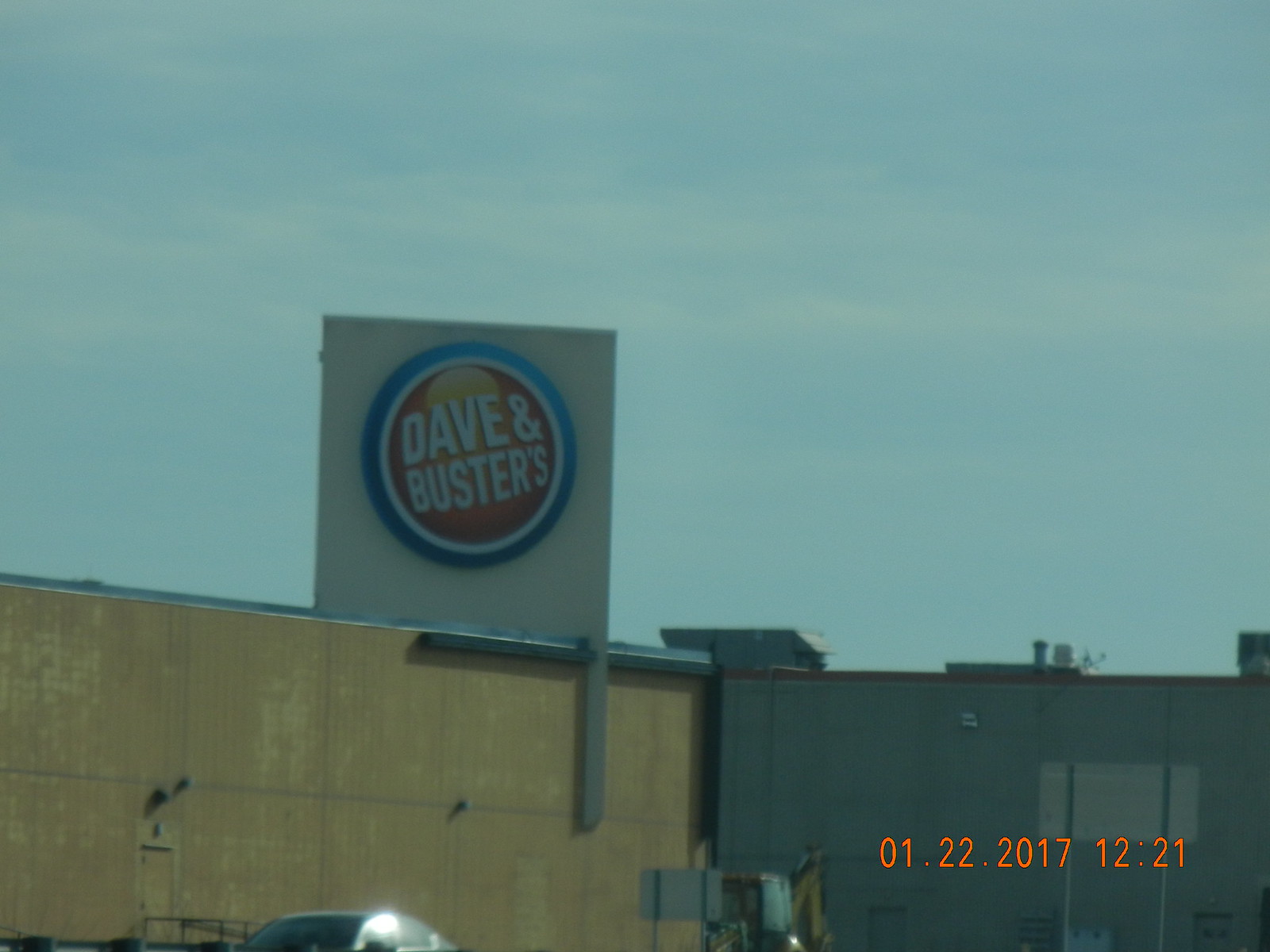The image depicts a slightly blurry and potentially scanned photograph of a commercial building complex. On the left, there is a lighter, dark tan building connected to a more angled, dark gray building. Atop the tan structure is a prominent white rectangular sign, featuring three circles: a blue one, a white one, and a shaded orangish circle with the "Dave & Buster's" logo in white. The reflection of a car from the parking lot is faintly visible on the building's surface, diffused by the bright sunlight. In the bottom right corner, the photo has a timestamp in orange lettering over the gray building, reading "01.22.2017" and "12:21". The sky is a light blue, adorned with a few distant white clouds, contributing to the overall sunny ambiance of the scene.